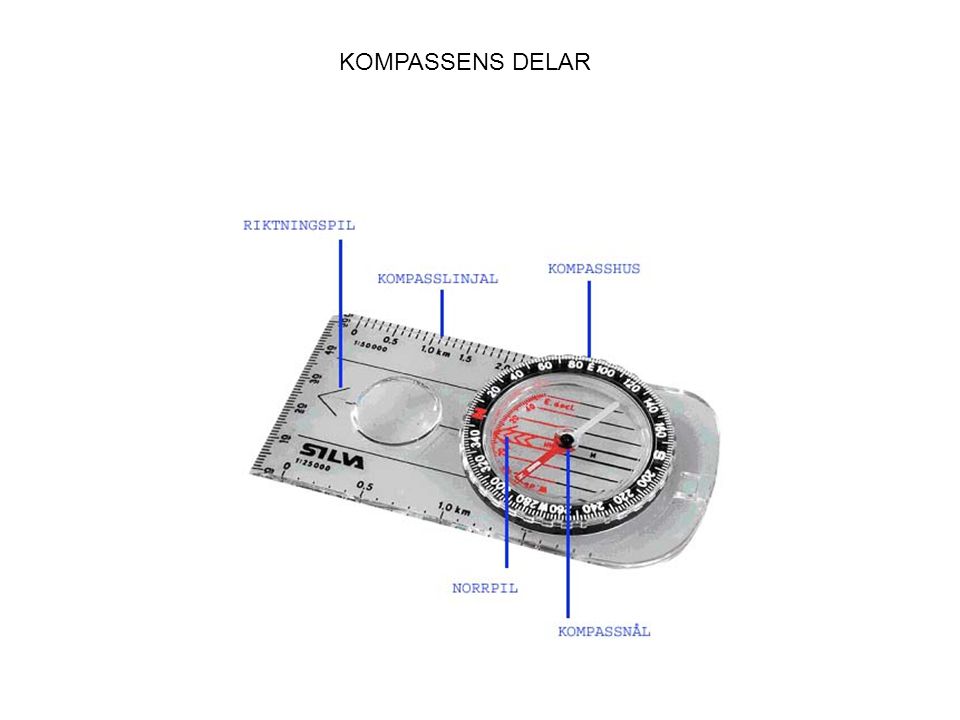The illustration depicts a detailed diagram of a measuring device, likely a compass, labeled in a foreign language. At the top, in fine black writing, it reads "KOMPASSENS DELAR." Below this heading, featured prominently on a white background, are several labeled components of the instrument. The compass itself is depicted as a thin, flat, rectangular silver object with black numbers resembling a ruler along the left and top edges. On the right-hand side of the device, there's a circular dial with a black background and white numbers, featuring a central white arrow. Radiating out from the compass are several blue lines pointing to different parts. These are labeled: "RIKTNINGSPIL" indicating an arrow pointing downwards, "KOMPASSILNJAL" referring to the measurement part, and "KOMPASSHUS" pointing to the compass settings. On the opposite side, "NORRPIL" denotes an arrow pointing north, and "KOMPASSNAL" marks the middle of the compass dial. In the bottom left corner, the word "silva" appears in black letters, suggesting the brand. Overall, the image combines elements of technical blueprint and instructional diagram to showcase the components and functionality of the compass.